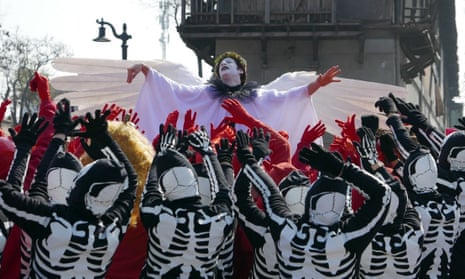The photograph captures a vibrant outdoor gathering, likely a theatrical or dance performance. At the center of the image stands a person dressed as an angel, visible from the midsection up. This central figure is adorned in a white robe with a black, ruffled collar and has their arms spread out to the sides, with hands open and slightly lowered. Their face is painted white with dramatic black makeup around the eyes and mouth, and they have short, curly brown hair. Large white wings extend from their back, giving them an ethereal appearance. The person gazes upwards with their head slightly tilted back.

In front of this angelic figure, a crowd faces the camera, with the bottom half of the image filled with raised arms. The majority of these individuals are dressed in black bodysuits decorated with white skeletal graphics, including bones on the arms and heads designed to look like skulls. Interspersed among these skeletons are several people in vivid red costumes, adding a stark contrast to the monochromatic skeletons.

In the background of the image, on the right side, there is a visible building, while on the top left, a pole with a bell and some distant trees can be seen, framing the scene.